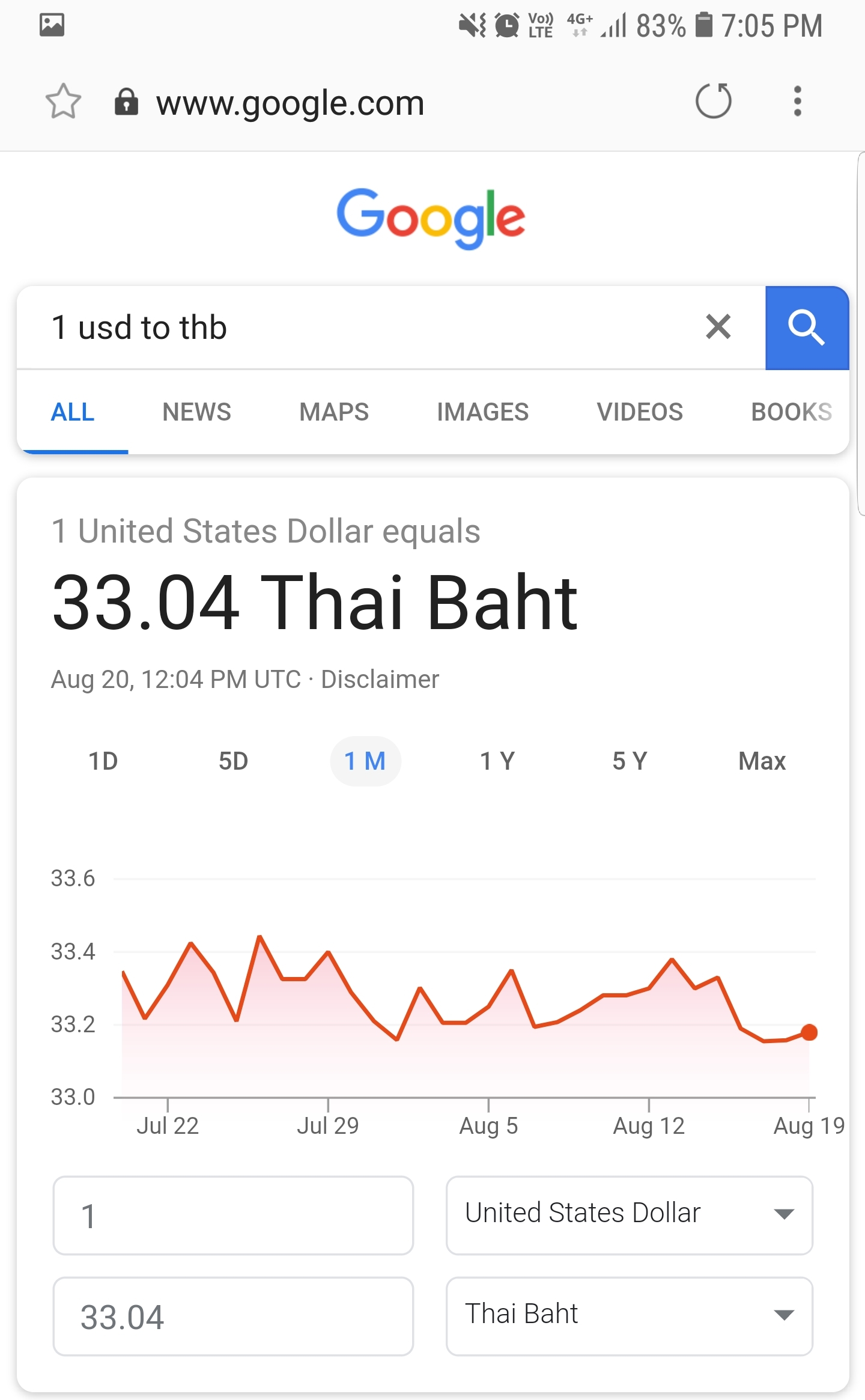A detailed smartphone screenshot captures a web page displaying the currency conversion rate from United States Dollars (USD) to Thai Baht (THB). At the top of the screen, typical Android status icons are visible, including a picture icon on the top left, a silent mode icon, a vibrate mode icon, an alarm indicator, signal strength bars, a battery level at 83%, and the time, 7:05 PM. 

The main content reveals the smartphone's browser interface. There's an unselected gray star, signifying the page is not bookmarked, and a lock icon next to the URL "www.google.com," ensuring a secure connection. To the right of the lock icon, there are a refresh icon and a three-vertical-dots menu icon for additional browser options.

The Google search bar shows the query "1 USD to THB," accompanied by a clear (X) button and a blue search button with a white magnifying glass icon. The search results are categorized into tabs: All, News, Maps, Images, Videos, and Books, with the "All" tab currently selected.

The main result indicates that "1 USD equals 33.04 THB" as of August 20th, 12:04 PM UTC, with a disclaimer note below. There are options to view historical data over different periods: 1 day, 5 days, 1 month (selected), 1 year, 5 years, and maximum duration. A graph below this information visualizes the exchange rate trends from approximately July 20th to August 20th.

At the bottom, input boxes allow users to convert different amounts. The first box displays "1 USD," and directly beneath it, another box shows "33.04 THB," with drop-down menus for selecting different currencies.

This detailed capture effectively serves users needing quick and comprehensive currency conversion details.